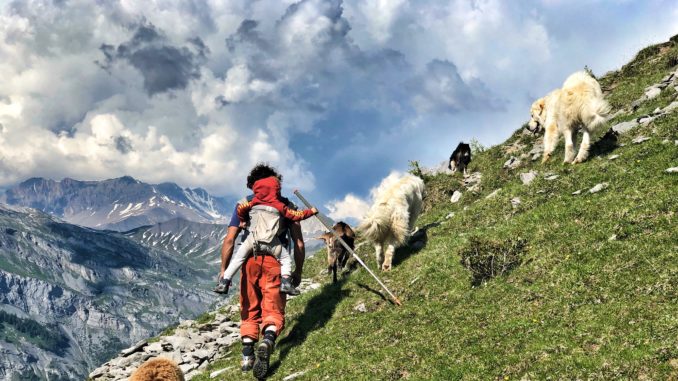The photograph captures a steep, green mountainside under a cloudy sky, where an individual, with a child wearing a red hood on their back, is accompanied by a group of approximately four fluffy, yellowish animals that resemble large sheepdogs. The person, dressed in blue and red clothing with black hiking boots, holds a long stick, possibly a hiking stick or a sword, angled downward as they lead the animals. The sloped, green grass terrain tilts to the right, hinting at the steepness of the hill. To the left, snow-capped mountains rise majestically in the background, partially obscured by large clusters of white clouds that hang suspended in the sky.